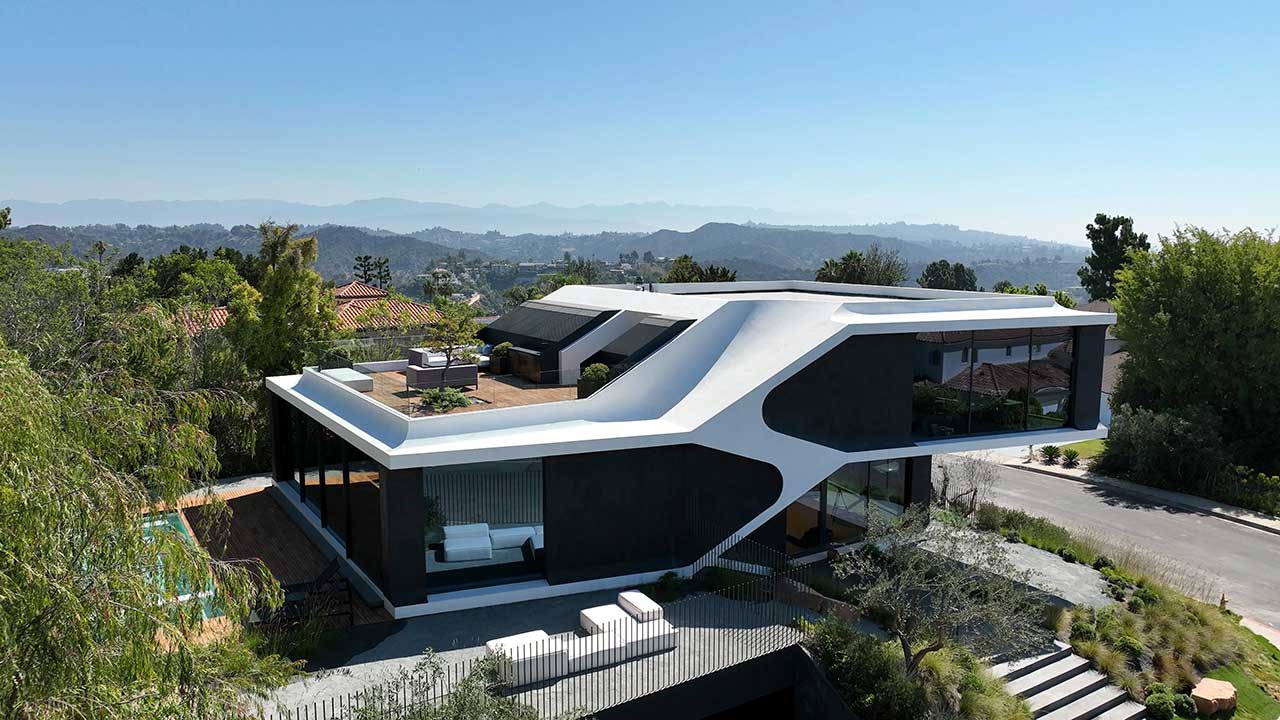This image showcases an extraordinarily futuristic, two-story home perched on a hilltop, likely in a sunny, scenic location reminiscent of California. The architectural design is marked by sleek white accents contrasted with black details, and incorporates extensive use of glass panels for most of the walls, giving it a distinctive, ultra-modern look. The structure intriguingly resembles two car CD consoles fused together and features large, expansive windows. 

The ground floor includes an inviting pool in the backyard, partially obscured by lush tree cover, and accompanied by a cozy lounging area complete with a white sofa on the side of the house. A sidewalk, flanked by steps rising from the street, leads to the entrance. The second floor boasts an outdoor deck that serves as a luxurious landscape lounging area, highlighted by a tree and more seating options. Towering above, it offers panoramic views of rolling hills, a bright blue sky, and occasional neighboring houses. A bar area is hinted at, complementing the overall opulent lifestyle conveyed by the home.